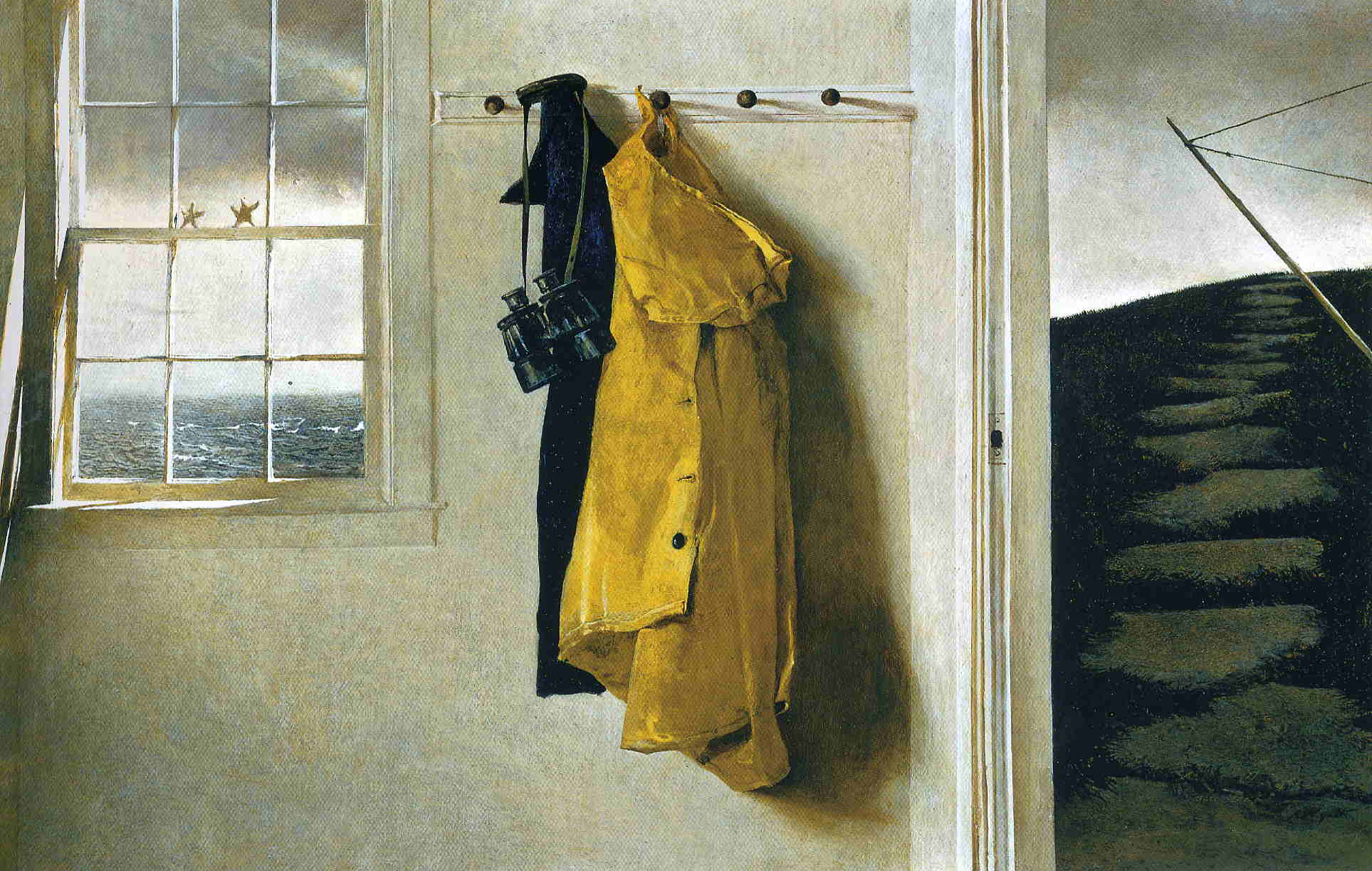The image is a painting by Andrew Wyeth titled "Yellow Coat." It depicts a hallway inside a house with a light beige cream-colored wall. The wall features a coat rack with five hooks, the second of which holds a heavily used yellow rain slicker with a hood, visible buttons, and buttonholes, as well as a pair of binoculars. The third hook holds a black, thinner jacket with no hood. The first, fourth, and fifth hooks are empty. On the left side of the painting, there is a closed multi-pane window adorned with two starfish in the center pane. Through the window, one can see a rough sea with choppy white waters under a cloudy, gray sky, indicating that the binoculars serve the purpose of observing the seaside. On the right side, an open doorway reveals flat stone pavers leading up to a dark hill, complemented by the outdoor light shining in, casting reflections and adding to the tranquil yet ominous seaside atmosphere. The predominant colors in the painting are yellow, white, blue, black, and tan.